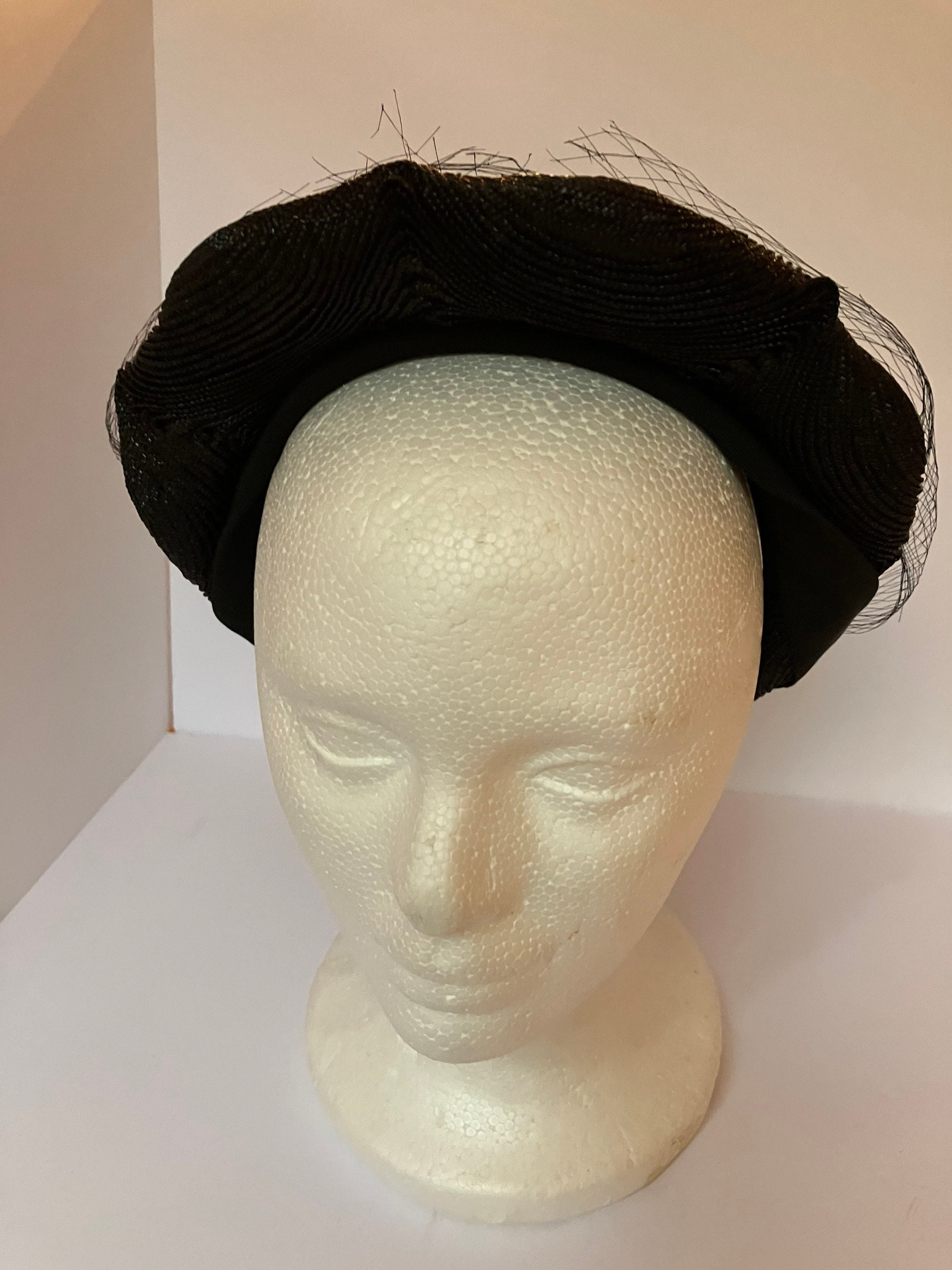The photograph features a vintage black hat resting on a slightly tilted, weathered styrofoam mannequin head. The head, which has basic facial features and a small neck base, is positioned within a white or very light pink cubicle-like compartment. The hat, potentially crafted from a straw-like or knit material, has a broad, wavy brim and is adorned with a frayed black netting akin to a veil, with noticeable tears around the top. The entire setup gives the impression of a product photo, possibly emphasizing the aged and delicate nature of the hat and its mesh detailing. The mannequin head faces the camera but tilts slightly to the left, and it is placed in the compartment's visible back-left corner, adding depth to the composition.